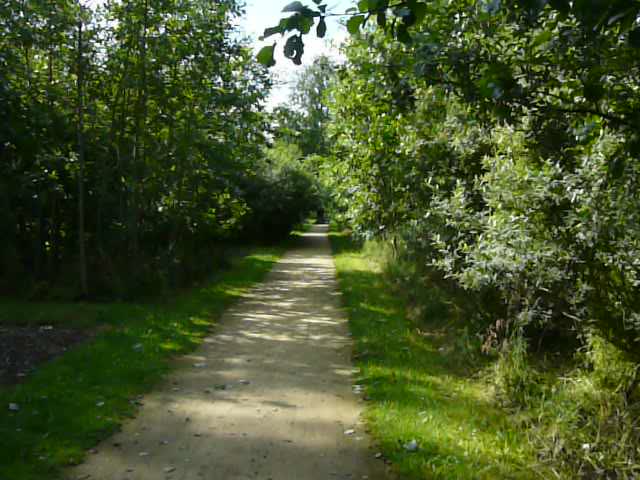The image depicts a serene and picturesque nature scene with a well-maintained walking path that begins at the bottom of the photo and extends into the center, vanishing into the distance. The path, light brown in color and seemingly made of compacted earth or concrete, is flanked on both sides by stretches of lush, green grass. The grass is neatly trimmed, albeit with some encroachment onto the trail, suggesting regular maintenance but also a touch of natural wildness.

On either side of the grass, dense foliage including trees and various plants adds depth and a sense of being enveloped by nature. This dense greenery forms an arching canopy over the trail in the distance, creating a tunnel-like effect that draws the eye further along the path. In the top corners, the foliage becomes taller and denser, framing the pathway and guiding the viewer's focus towards the vanishing point. 

Above the scene, a partly cloudy sky peeks through, the blue and white hues adding a soft contrast to the greens and browns below. The sky's gentle illumination indicates a clear daytime setting. Scattered leaves on the trail hint at the early stages of autumn, adding a touch of seasonal change to the vibrant greens of the grass and trees. The overall atmosphere is one of peaceful, natural beauty, as if inviting a leisurely walk or bike ride through this idyllic forested area.